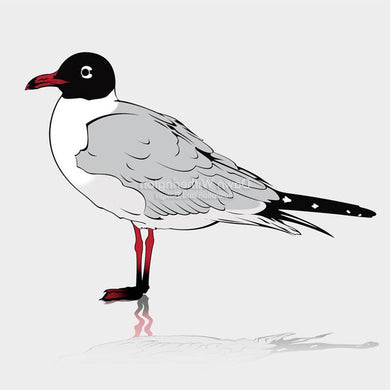This artwork, a pen and ink drawing with hints of paint, vividly portrays a bird on a light gray background. The bird stands, casting a faint shadow below, possibly on water or ice. It faces sideways, revealing a striking black head with a long orange-ish, reddish beak. Its eyes are gray with black pupils. The bird's chest is white, blending seamlessly into its lighter gray wings marked by visible feathers. Its tail feathers are black. Thin, spindly orange legs support the bird, ending in black webbed feet. The subtlety of the piece is enhanced by faint, blended text on the bird's body, reading "Down, Washington," imbuing it with an extra layer of hand-painted artistry.